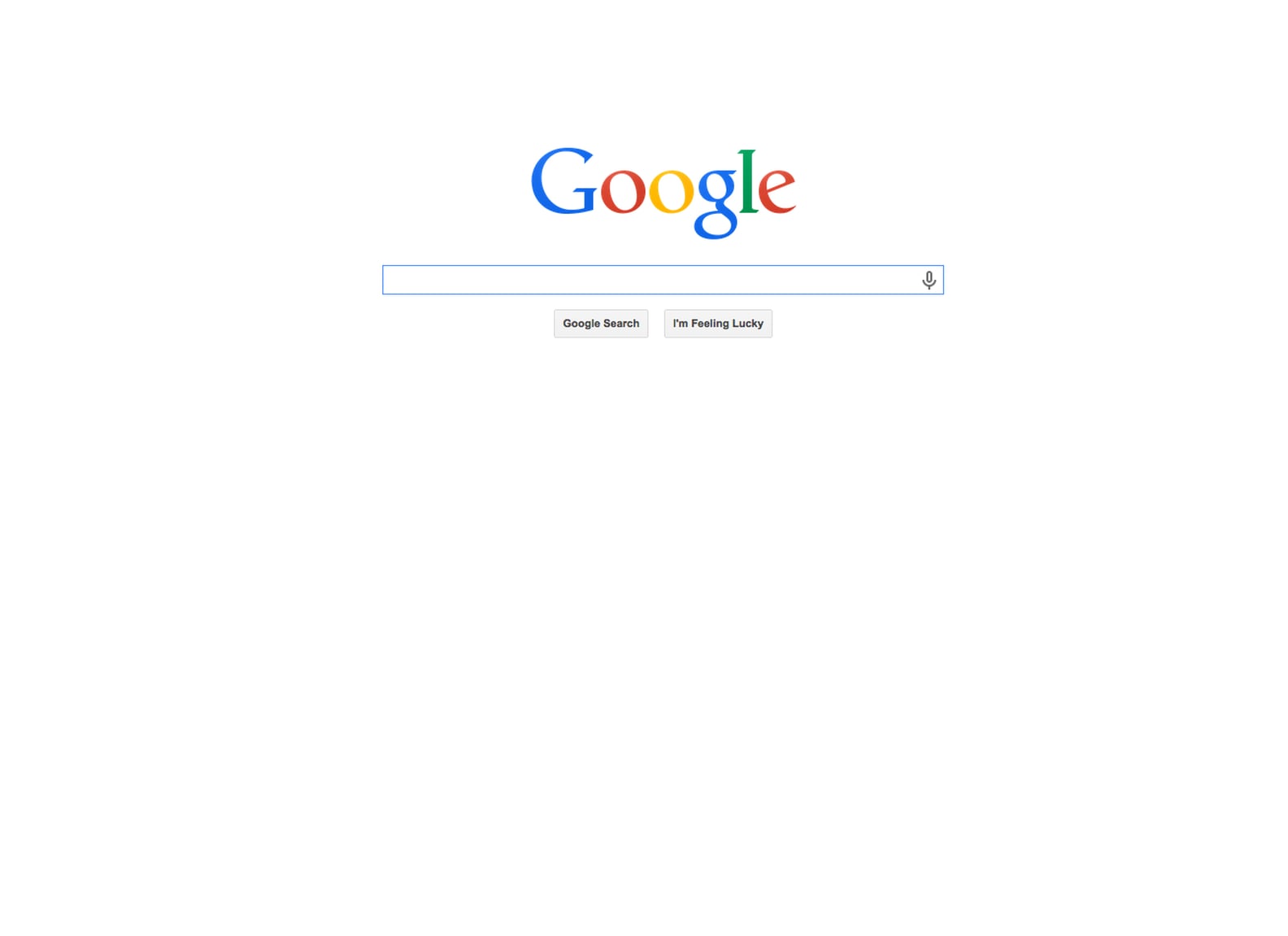The image displays the minimalistic home page of Google. The background is a clean, stark white, creating a clear and uncluttered space. Centered at the top is the iconic Google logo, with each letter rendered in its distinctive colors: the first "G" is blue, the first "O" is red, the second "O" is yellow, the second "G" is blue, the "L" is green, and the "E" is red.

Beneath the logo sits a rectangular search bar with a subtle light blue border. The interior of the search bar is white, and positioned on the far right inside the bar is a black microphone icon, indicative of Google's voice search functionality.

Directly below the search bar are two rectangular buttons. The button on the left reads "Google Search," while the button on the right reads "I'm Feeling Lucky." Both buttons feature black text on a light gray background, maintaining the simple and user-friendly design that Google is known for.